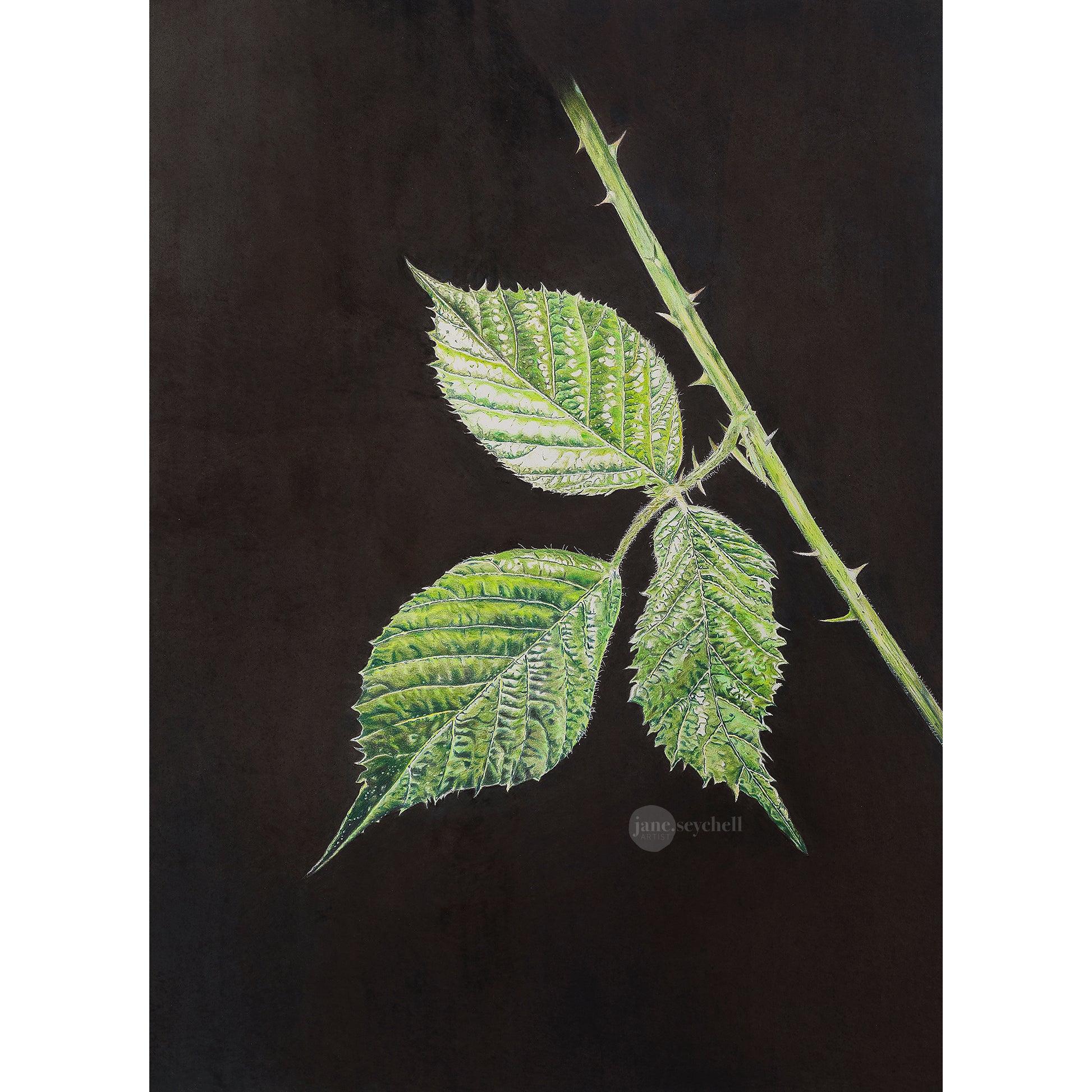This photograph captures a vividly lit green branch of a blackberry bush against a completely black background. The prominent thorny stem angles from the top center to just below the right center of the image. Branching off from this stem is a smaller stem, also dotted with thorns, which supports three large, distinct green leaves characteristic of a blackberry plant. The luminous quality of the bush contrasts sharply with the darkness surrounding it, accentuating the prickly details of the thorns and leaves. Beneath the plant, there is a subtle watermark in gray letters that reads "Jane Seychell."